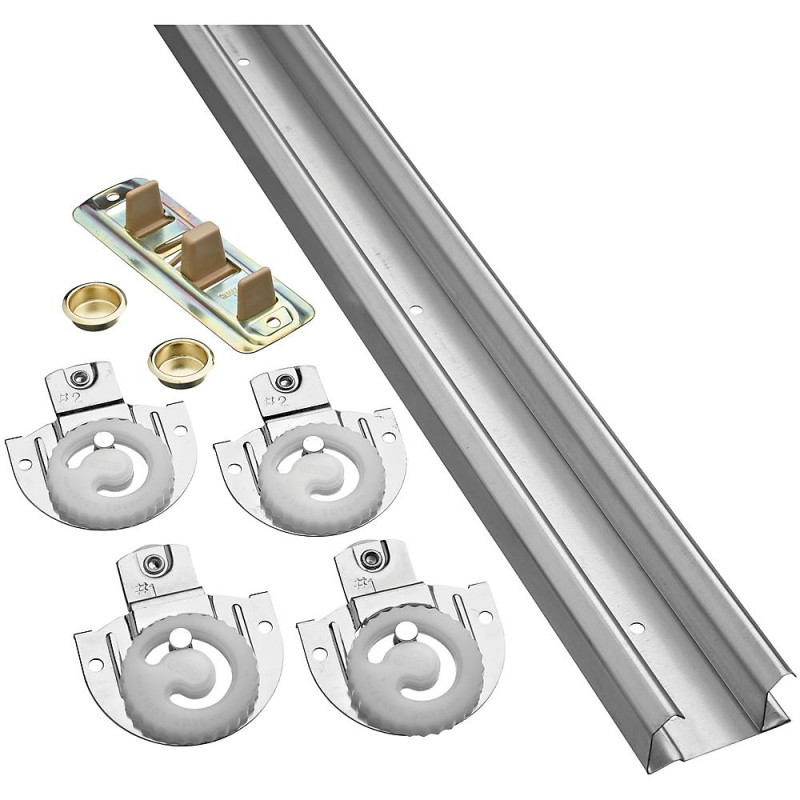The photograph features a detailed hardware locking mechanism. Central to the image is a straight metal slide with two hooks running down its length, flanking a flat metal area between them. To the left of this metal slide, there are four identical white plastic rings with nails in their centers, attached to a flat metallic base. Additionally, there are two small gold thumbtacks below a rectangular gold piece that has four brown rectangular plastic tabs protruding from it. These components appear to be part of a system meant for repairing or assembling a piece of furniture, such as a dresser drawer.